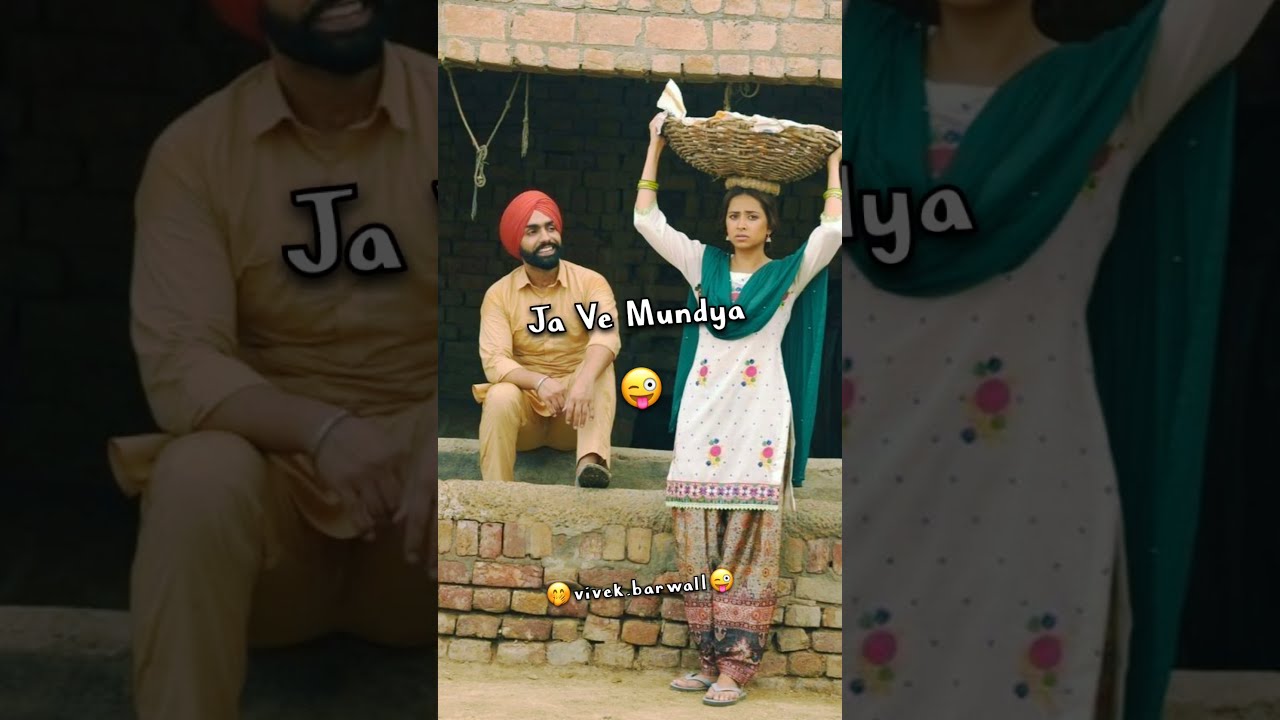In the center of this horizontal image, a woman stands with a large, round brown wicker basket balanced on her head. She has dark hair pulled back, and she's dressed in an ensemble that includes a long, white and pink-patterned top with flowering dots, baggy patterned pants, flip-flops, and a green scarf draped around her neck. Her facial expression is neutral, and she leans slightly against a waist-high stone retaining wall with a dirt ground beneath her. To her left, a man sits on the stone wall wearing a red turban, a beige or yellowish outfit consisting of a top and pants, and flip-flops. He has a black mustache and beard and is smiling at her with his mouth open. Above them, the background is created by faded close-ups of their faces; the left side shows a partial close-up of the man with “JA” written, and the right side shows the woman with “LYA”. Across the main image, white text reads “JAVE MUNDYA.” A cheeky smiley face emoji with a tongue sticking out is placed between the two central figures. The backdrop also reveals partial brick walls, adding to the rustic ambiance.